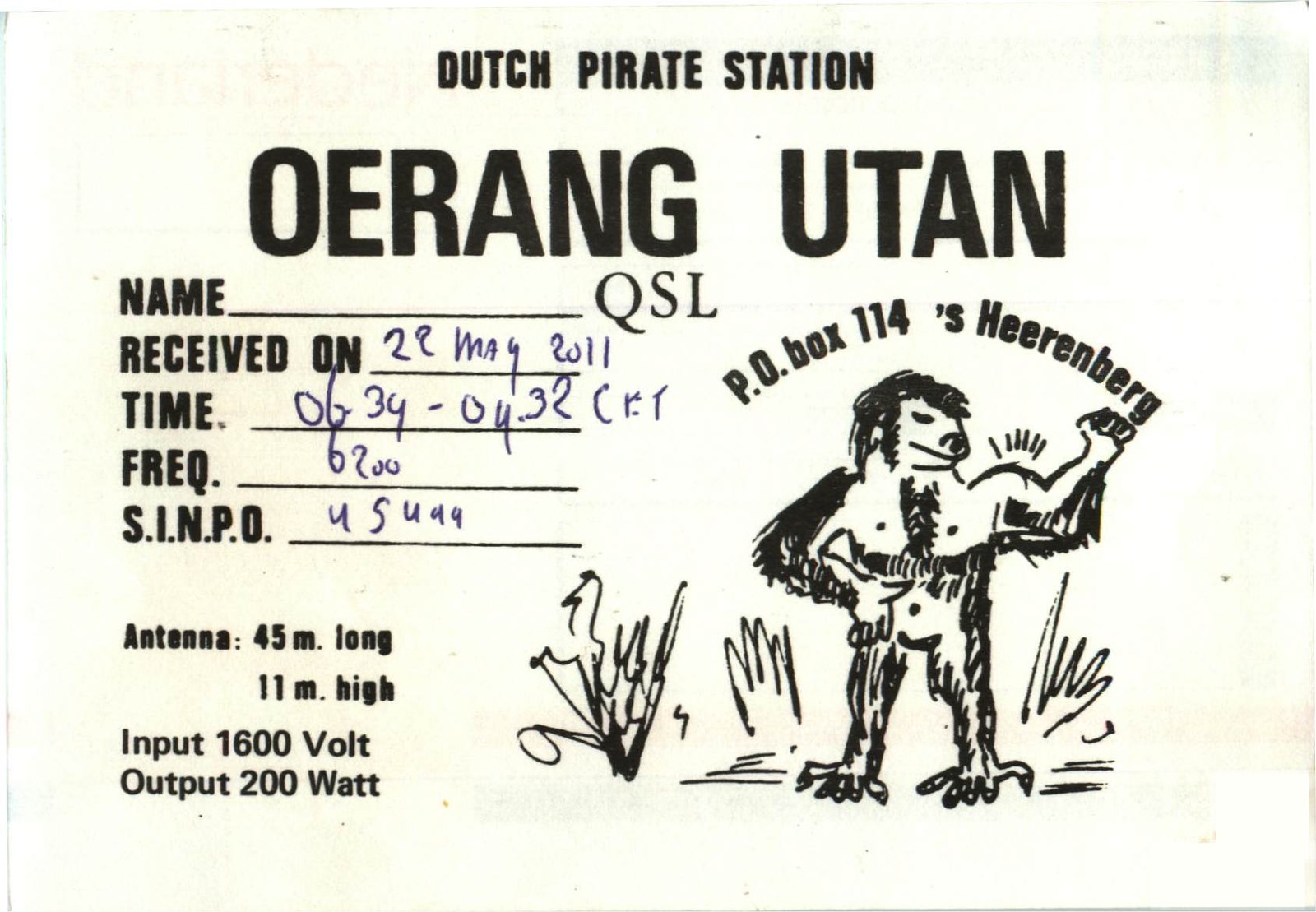This image depicts a square business card titled "Dutch Pirate Station" at the top in bold black letters, with the largest text being "OERANG UTAN" in all capital letters beneath it. The card includes a section filled out by hand with the following details: the name is listed as QSL, which was received on 29 May 2011, penned in blue ink. The time is recorded as 0634 to 0432 CET, although the handwriting appears somewhat sloppy. The frequency (FREQ) is indicated as 6200, with the signal quality (SINPO) marked as 45499. Additionally, antenna specifications are detailed, noting it is 45 meters long and 11 meters high, with an input of 1600 volts and an output of 200 watts. On the right side of the card, there is a cartoonish illustration resembling a caveman or ape with an abstract appearance. Above this figure, the text "PO Box 114 S Hirenburg" is displayed.